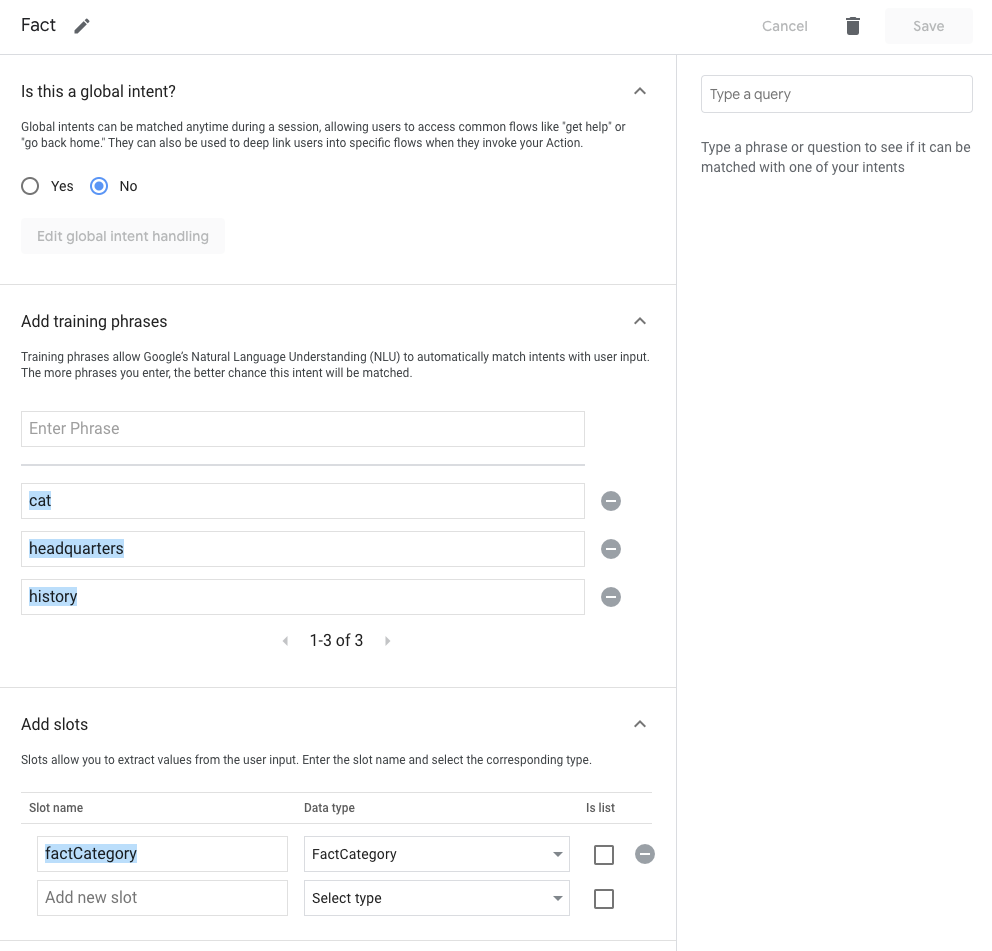This image depicts a detailed screenshot of a user interface for configuring global intents and training phases in a conversational AI or chatbot development platform.

At the top of the page, there is a section labeled "Fact" alongside an icon resembling a crayon. Beneath this, a prompt asks, "Is this a global intent?" It explains, "Global intents can be matched anytime during a session, allowing users to access common flows like 'get help' or 'go back home.' They can also be used to deep link users into specific flows when they invoke your action." The options provided are represented by circles labeled "Yes" and "No," with the "No" circle filled in blue. Below this section, there's a faded, shaded text that reads "Edit global intent handling."

The second section is titled "Adding Training Phrases." It explains, "Training phrases allow Google's natural language understanding to automatically match intents with user input. The more phrases you enter, the better chances intent will be matched." Below this instruction, there is an empty input box labeled "Enter Phrase."

Further down, there's a section titled "Cat Headquarters History," each placed within its own blue-highlighted box. Each box has a grey circle with a white minus sign next to it, suggesting the option to remove these entries.

The final section is labeled "Add Slots." This part instructs the user on how to extract values from user input. The instructions read, "Enter the slot name and select the corresponding type." Below this are fields labeled "Slot Name" and "Data Type." A list displays "Fact Category," highlighted in blue, followed by an empty text box and a grey circle with a white line. Additionally, there are options labeled "Add New Slot," "Select Type," with accompanying drop-down menus and empty input fields to enter values.